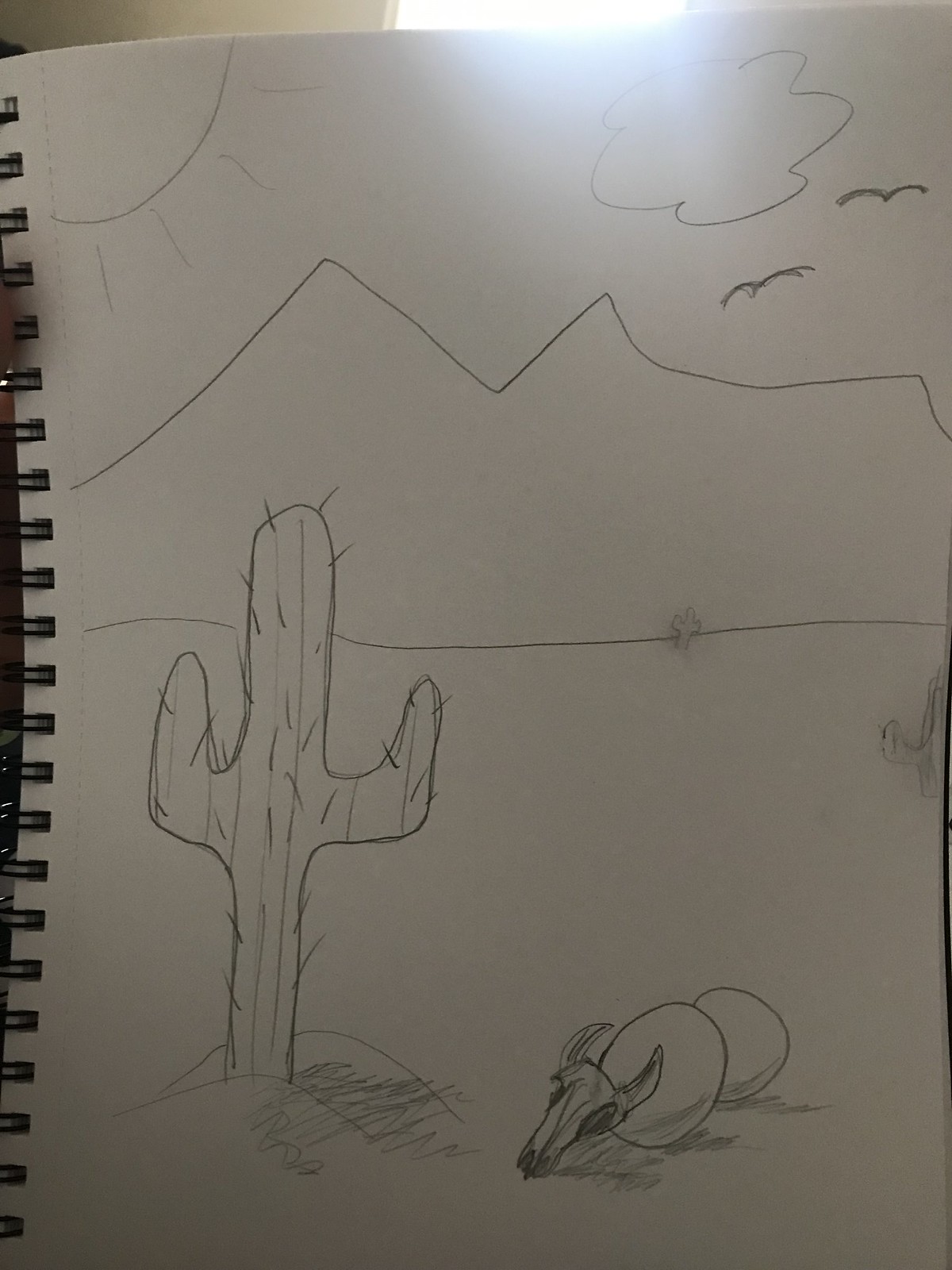In a black spiral-bound sketchbook with plain white paper, one can find a detailed pencil drawing that likely belongs to a child, possibly created in an art class. The scene is set in a rudimentary style, characteristic of early artistic attempts. In the top right corner, a sun emanates light with expressive rays, while a cloud floats to its left. The sky features two simplistic bird outlines hovering just left of the sun. Below, a jagged mountain range stretches across the background, creating a natural horizon. Dominating the foreground is a spiky cactus, its surface dotted with needles and casting a noticeable shadow. Adjacent to the cactus lies the detailed skeleton of a steer's head, largely intact, accompanied by two sizable boulders. The drawing contains minor smudges, possibly evidence of the artist's learning process, suggesting they followed a learn-to-draw guide. The entire scene, devoid of color, encapsulates a desert landscape with precision and thoughtful elements.